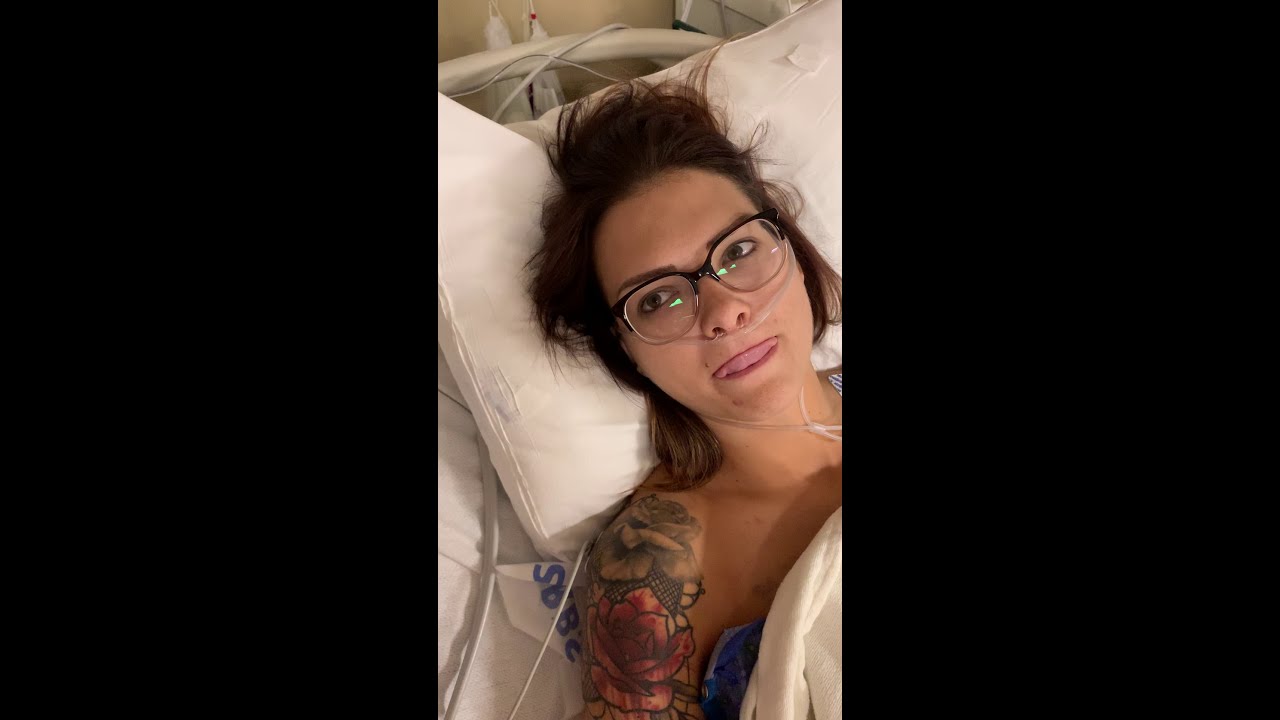This image features a vertical, rectangular photograph of a woman lying in a hospital bed, framed by thick black borders on the sides. The woman, appearing to be in her late 20s or early 30s, has messy, shoulder-length brown hair and wears eyeglasses with black or brown rims. She gazes directly at the camera with her brown eyes, her tongue slightly sticking out, touching her upper lip. She appears to be topless, with a white blanket or sheet partially covering her chest in the lower right corner. Her right arm displays a detailed floral tattoo in red and black, featuring a black rose and a red rose, with a small image of a couple dancing on top of the red rose. Medical equipment surrounds her: gray wires are visible to her side, and a clear tube runs into her nose, wrapping around her neck and extending behind her head. Additional cords are seen attached to a white bed frame behind her, draping down and off the sides of the image.